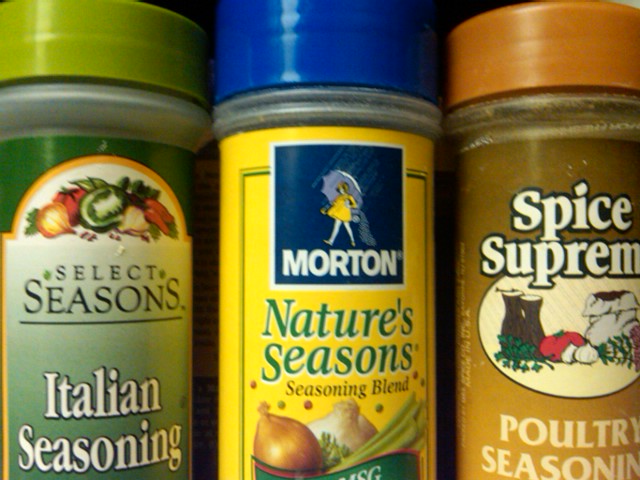The image depicts three plastic spice containers lined up closely together, partially cropped. 

On the left, there's a clear bottle with an olive green cap. The label is green at the top, featuring various vegetables, followed by the text "Select Seasons" in black, underneath which it says "Italian Seasoning" in white, outlined in black.

In the middle, there's another clear container with a blue cap. This bottle has a yellow label displaying the iconic Morton logo of a girl holding an umbrella against a blue background, outlined in white. Below the logo, it says "Morton" in large white print. The label continues to read "Nature Seasons" in green and "Seasoning Blend" in black, accompanied by images of garlic, onion, and green herbs.

On the right, there's a clear brown plastic container with an orange lid. The label is brown, outlined in white or puffy black letters, and reads "Spice Supreme" followed by "Poultry Seasoning" in a cream color. The label also features an oval filled with images of various vegetables, such as garlic and tomatoes.